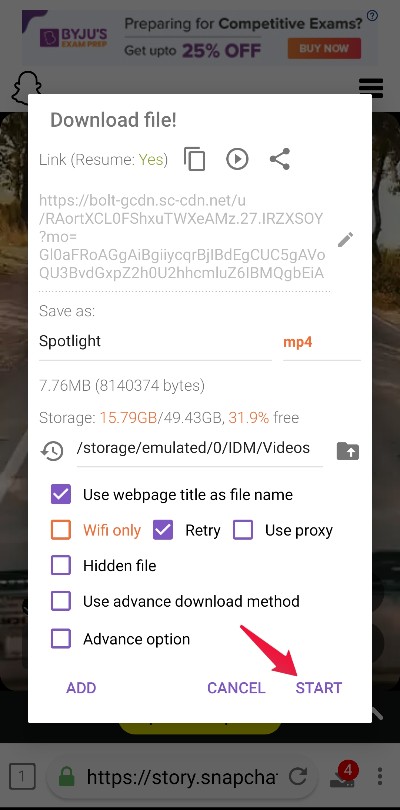This detailed caption provides a thorough description of the image:

---

The image is a screen capture of a mobile browser displayed in an unusual orientation, with the URL bar located at the bottom of the screen, likely due to user customization. The primary focus of the screen capture is a pop-up window which has grayed out the background, indicating an active dialog box.

Behind the pop-up, the website appears to be related to preparing for competitive exams, featuring a promotional banner that advertises up to 25% off with a 'Buy Now' call-to-action. The website also displays the Snapchat logo and a footer mentioning "story.snapchat," suggesting that the browser window might have been launched from within the Snapchat app.

The pop-up window dominating the image prompts the user to download a file. It includes the following elements:

- A prominent message saying, "Download file," with options "Resume" and "Yes."
- Multiple icons for additional actions: a share icon, a copy icon, and a play icon.
- A lengthy URL displayed under the download prompt.
- A file name input field labeled "Save as: spotlight.mp4," with ".mp4" highlighted in red.
- Basic information about the file size, available storage on the user's device, and the editable storage path indicated with a file icon.
- Three checkboxes at the bottom of the popup, with black text and purple checkboxes. The checkboxes fill in with a white checkmark on a purple background when selected. The checked options in this image are:
  - "Use web page title as file name"
  - "Retry"

This detailed description encapsulates the visual and informational content of the screen capture.